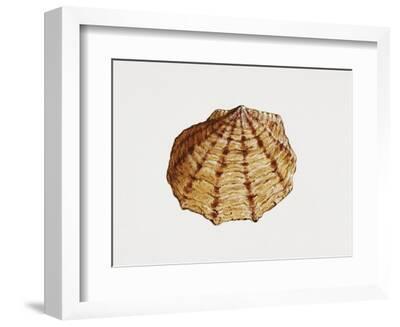The image is a framed art piece featuring a detailed depiction of a light brown seashell, likely a clamshell or oyster shell. The shell is centered within the artwork and displayed against a white background, which extends through a white mat and into the surrounding white frame. The shell is illustrated with downward striations that are slightly darker brown, adding realistic texture and shading, particularly on the left side. The simplicity of the composition, with the creamy white background and singular shell, creates a minimalist aesthetic. The art piece itself is neatly bordered by a small black line, followed by a white margin, and encased in a freestanding white frame.